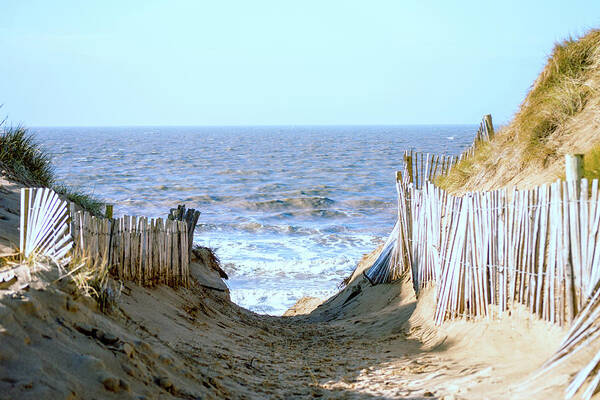This image captures a picturesque beachfront walkway leading from an access area down to the ocean. At the forefront, a well-worn sandy path meanders through the scene, stretching from the upper left to the lower middle before opening up onto the beach. This path, characterized by numerous footprints, hints at frequent use by beachgoers heading towards the inviting, crystal-like blue water. 

On either side of the path are dunes adorned with tufts of seagrass, adding a splash of green to the predominantly sandy landscape. These dunes rise gently from the walkway, forming natural barriers that help contain the shifting sands. Flanking the path, a pair of aging reed snow fences stand—one on each side—constructed of thin, weathered wooden slats, their white and tan hues blending into the earthy surroundings. These fences, though somewhat rickety and leaning in spots, serve the essential function of stabilizing the dunes.

The horizon stretches out beyond the dunes, where the calm blue sky meets the equally blue ocean. The water exhibits gentle waves that gradually build to soft, foamy crests as they approach the shore. The overall scene combines natural beauty with evidence of human interaction, creating a serene but dynamic coastal landscape.